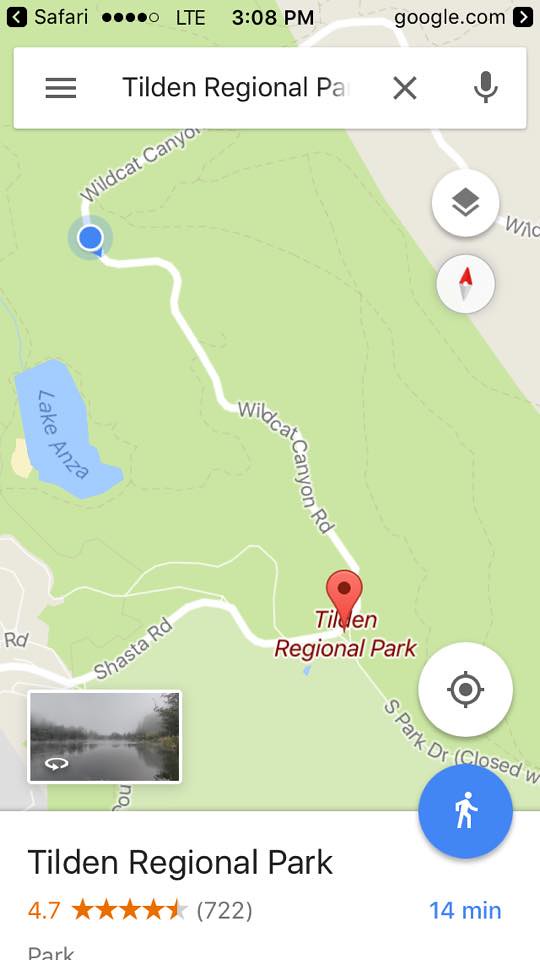This image is a screenshot taken from a mobile device depicting GPS directions, likely from Google Maps accessed through Safari browser. The screenshot was captured at 3:08 PM and prominently displays information about Tilden Regional Park. The park has a rating of 4.7 stars from 722 reviews, with the stars rendered in bright orange, including four full stars and a partial star.

The map in the center of the screenshot is predominantly light green, with Tilden Regional Park marked in red, featuring a red location pin. To the left of the park, a light blue lake, labeled "Lake Anza" in dark blue text, is visible. Another point of interest, "Wildcat Canyon," is marked above the lake with a blue marker.

At the bottom portion of the screenshot, the text "Tilden Regional Park" appears on a white background in black text. The right side of the image indicates that it takes approximately 14 minutes to reach the park, either by driving or walking.

Additionally, the presence of "google.com" on the right side of the screen further suggests that this information is being viewed through Google Maps.